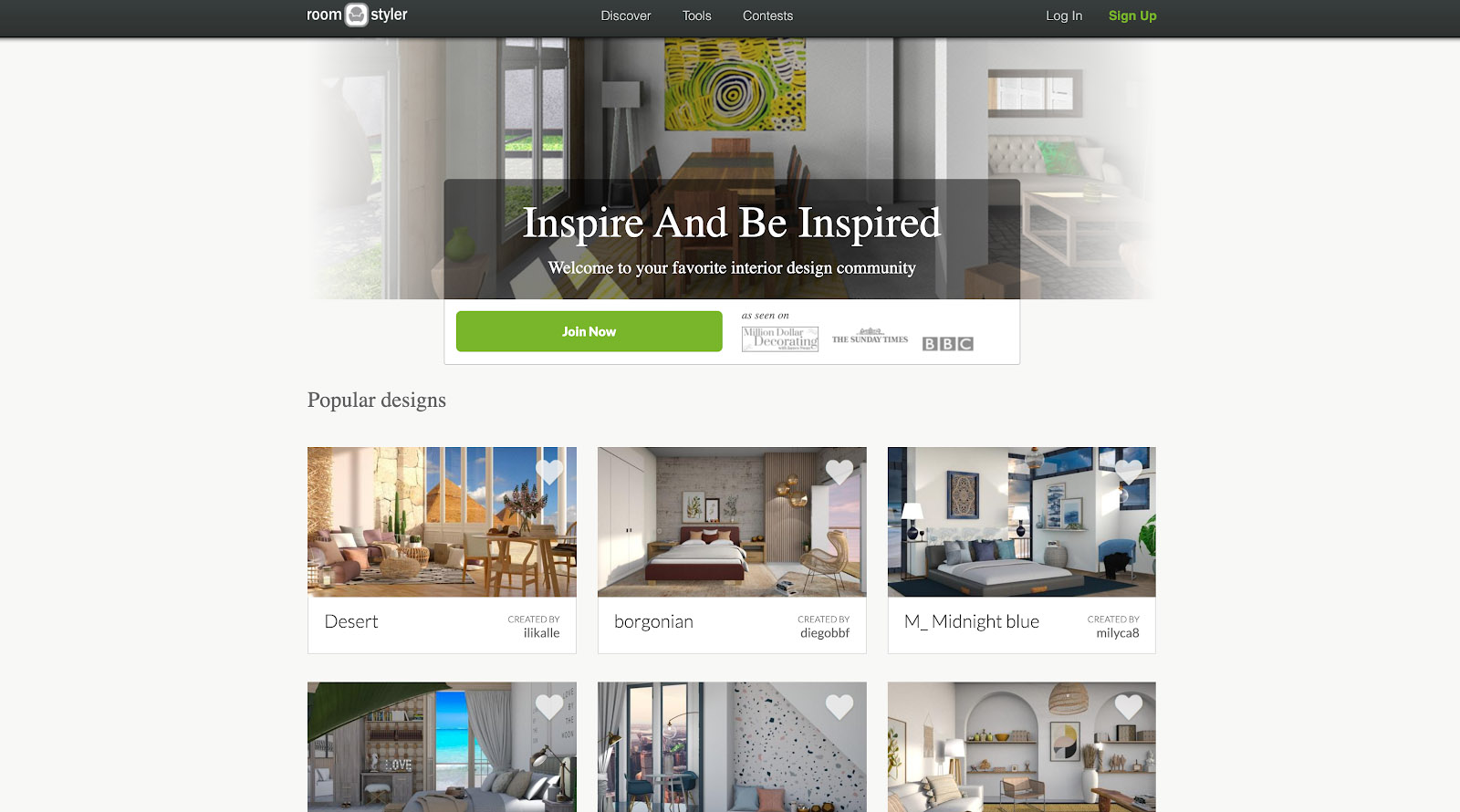This screenshot captures the elegant interface of the RoomStyler website. At the very top, a sleek gray navigation bar features three primary tabs: "Discover," "Tools," and "Contests." On the right side of this bar, there are two buttons for user accounts: a gray "Login" button and a green "Sign up" button, inviting new users to join.

Just below the navigation bar, a captivating banner image showcases a tastefully decorated living or dining room with a neutral color palette accentuated by pops of color. The room features light gray walls and windows, a central wooden table and chair set perched on a beige rug, and cozy seating to the right, including couches and a box with a green pillow. A vibrant artwork featuring green, yellow, and black and white dominates the wall above the dining set.

Overlaid text on the banner image reads, "Inspire and be inspired. Welcome to your favorite interior design community," creating a warm and inviting atmosphere. Beneath this welcome message, a prominent green "Join Now" button encourages visitors to become part of the community. Adjacent to this call-to-action is a smaller section highlighting media mentions, stating "As seen on" followed by the logos of "Million Dollar Decorating," "The Sunday Times," and "BBC."

Further down, a section titled "Popular Designs" showcases six design thumbnails. The visible top three designs are named "Desert," "Argonian," and "M_Midnight Blue," each accompanied by its respective image. The bottom three designs, while partially visible, have their names cut off in the screenshot.